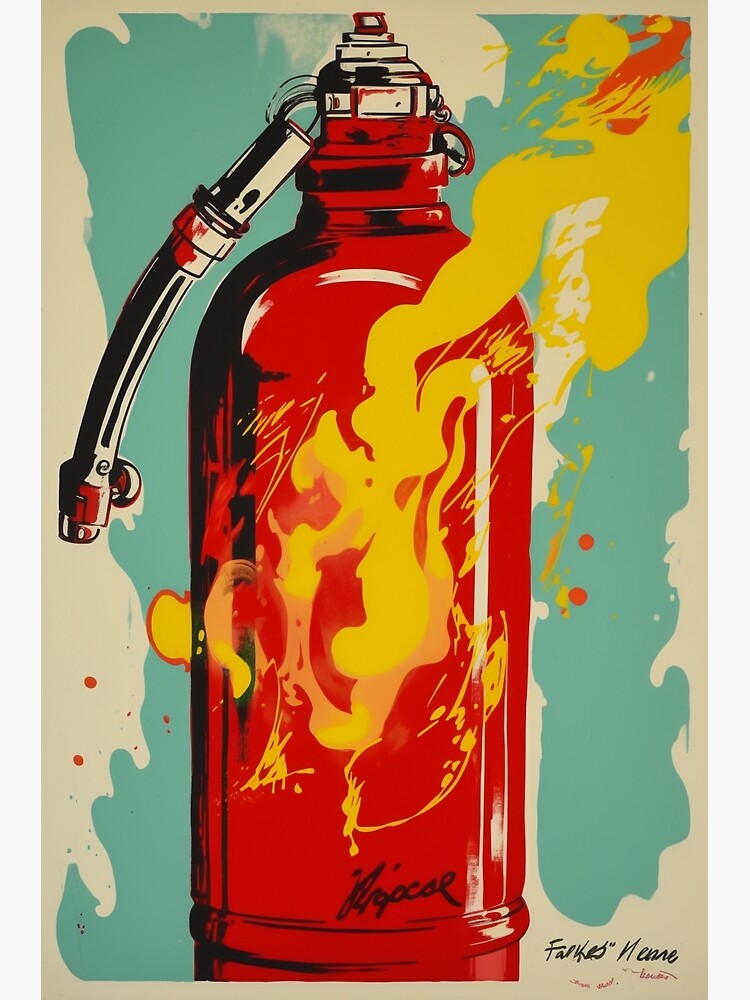This vintage-inspired poster features a central, striking illustration of a red fire extinguisher adorned with intricate black shadows and white highlights to emphasize its three-dimensional, cylindrical shape. The top of the extinguisher showcases a meticulously painted mechanism in white, representing the silver components, while the hose is carefully detailed with black wire and a curved nozzle accented with red reflections. The chaotic yet vibrant background—a splash of teal blue intermixed with dots of red and yellow paint—creates a dynamic canvas, enhancing the vibrant red of the extinguisher. Unique to the artwork is an overlay of yellow and red spatter that adds a fiery, almost surreal quality, particularly vivid in the upper right corner. The bottom right corner bears an artist's signature which appears to be "FALK NEME" and other indistinguishable red writing, hinting at authenticity and the artist’s personal touch. This piece, reminiscent of vintage advertisement posters, artfully combines elements of chaos and precision, making it a captivating visual experience.